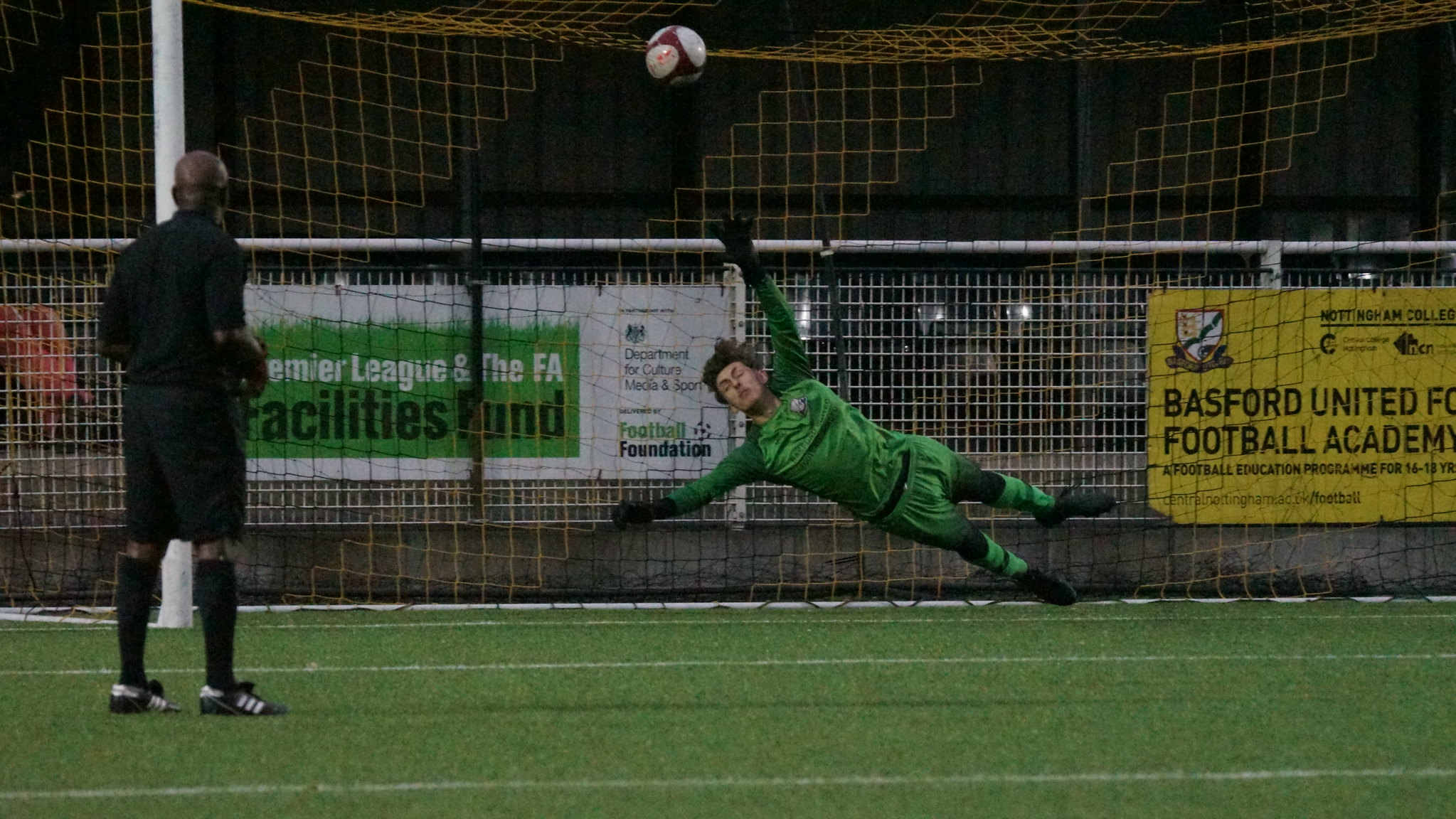This detailed photograph captures a dynamic moment in a soccer game, where a goalie dressed in a green uniform with black accents—long-sleeved shirt, gloves, knee braces, and shoes—is attempting a dramatic save. The goalie is suspended in midair, his body slanted with his feet closer to the ground and his arms stretched toward the ball, which hovers about two feet above him and appears to be heading towards the goal. The soccer ball itself is white and brown. Behind the goalie is the soccer net, obscuring the background except for a series of banners. Prominently displayed are advertisements that include a yellow billboard reading "Basford United Football Academy" and a green sign with "Premier League and FA Facilities." To the left of the frame, a referee, attired in an all-black uniform, closely observes the action. The scene is set on lush green turf, giving the impression of a well-maintained soccer pitch. The image conveys the intensity and athleticism of the match despite the empty stands, highlighting the well-branded and organized nature of the game.